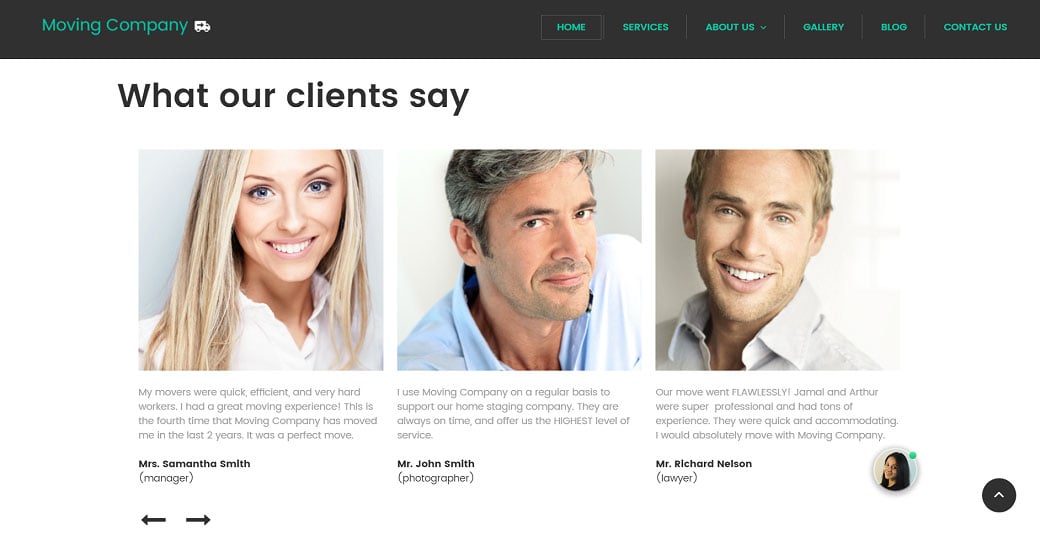The rectangular image features a long horizontal orientation. At the top, a black banner stretches from left to right, with "Moving Company" written in green letters, accompanied by a small symbol of a van to the right of the text. Below this banner, closer to the center, there are green text labels reading "Home," "Services," "About Us," "Gallery," "Blog," and "Contact Us," also in green.

The main background of the image is white. Centered prominently in black text, it reads "What Our Clients Say." Below this heading are three testimonial sections, each featuring an image and accompanying text.

On the left, there's a picture of a middle-aged white female. Her testimonial reads:
"My moves were quick, efficient, and the movers were very hard workers. I had a great moving experience. This is the fourth time that Moving Company has moved me in the last two years. It was a perfect move. - Miss Samantha Smith."

In the middle, there is a picture of a middle-aged white male. His testimonial reads:
"I use the company on a regular basis to support our home staging company. They are always on time and offer us the highest level of service. - Mr. John Smith."

On the right, there's a picture of another middle-aged white male. His testimonial reads:
"Our move went flawlessly. Jamal and Arthur were super professional and had a ton of experience. They were quick in accommodating. I would absolutely move with Moving Company again. - Mr. Richard Nelson."